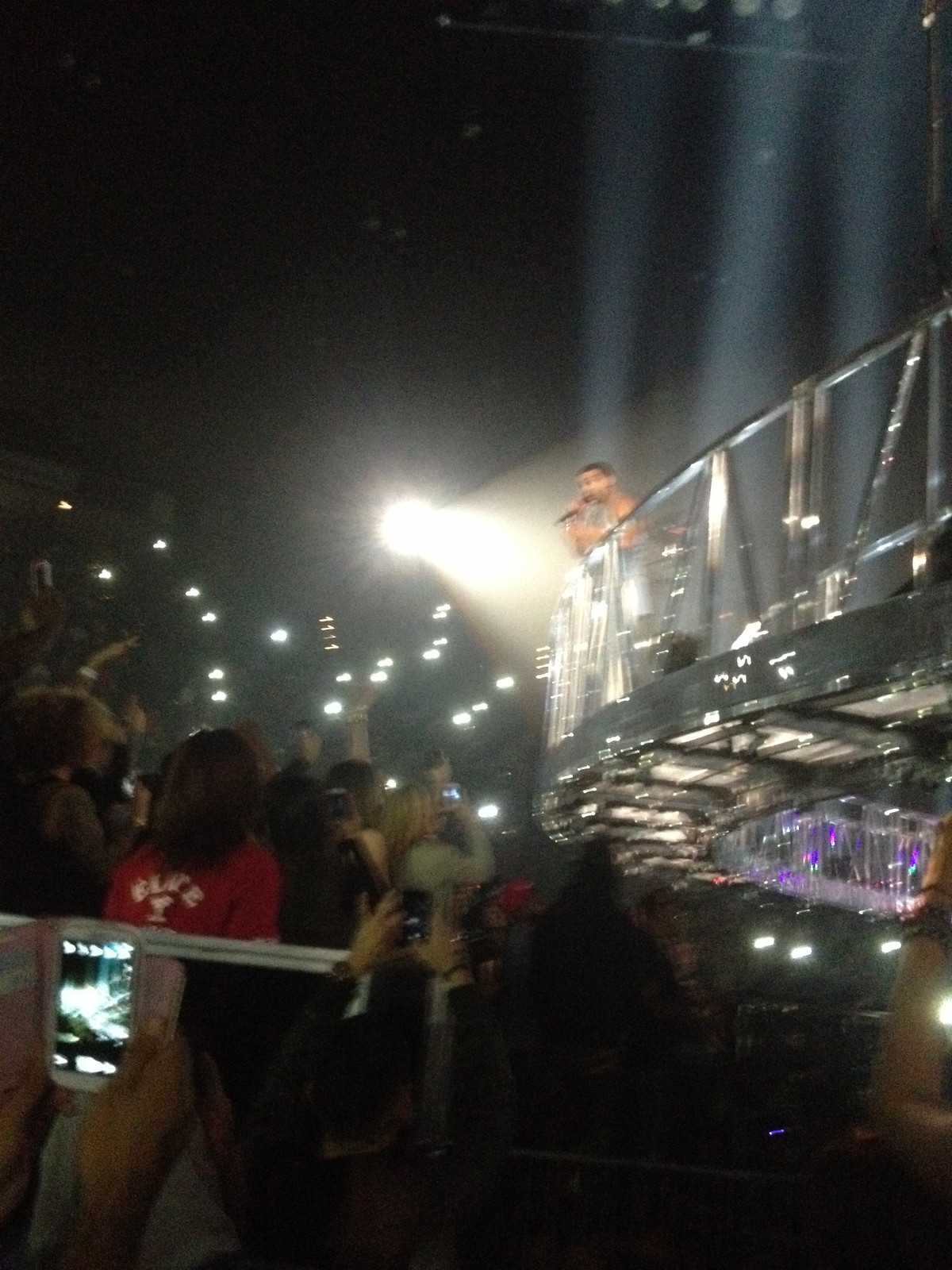In this photographic image set indoors at a nightclub or possibly outdoors in a stadium, a blurry figure of a black man is captured standing on a metal, grey bridge, elevated above his fans. The man, who could resemble popular singers like Jason Derulo, Drake, or Usher, is spotlighted from behind, creating a striking contrast with his surroundings. He wears a short-sleeved shirt and is engaged with a microphone, either singing or speaking as he looks down. From beneath the bridge, adoring fans, indistinct due to the blur, gaze upwards. Notably, one fan wears a red shirt with white lettering, possibly reading "EL" and "Z," while another in a white shirt looks on. Surrounding him, a sea of cell phone lights illuminates the atmosphere, creating a dynamic interplay of light. The stage, which appears to be a suspended circular metal platform with grating along the bottom, has a purple-lit structure underneath. The bottom right-hand corner of the image is shrouded in darkness, adding to the dramatic effect of the scene.